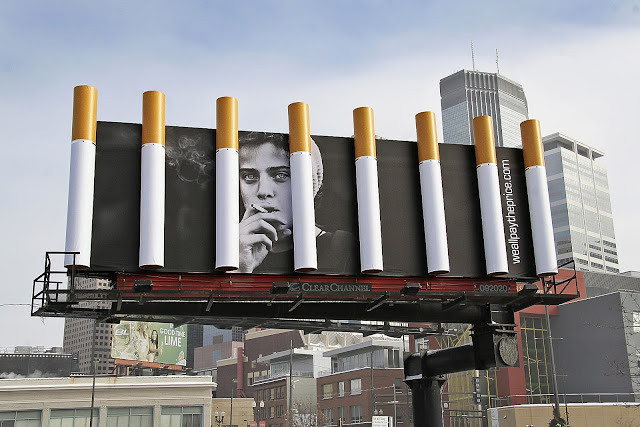This striking anti-cigarette campaign billboard, set against an urban backdrop, features a black-and-white image of a woman with a neutral expression as she smokes. The grayscale tones of her portrait underscore the somber message. The campaign's message, "we all pay the price.com," is prominently displayed in a vertically rotated font on the right side of the billboard. Adding a three-dimensional element, eight meticulously aligned giant cigarettes protrude from the billboard, symbolizing the intrusive nature of smoking. The background reveals a cityscape with numerous buildings, suggesting the pervasive reach of smoking and its societal impact.